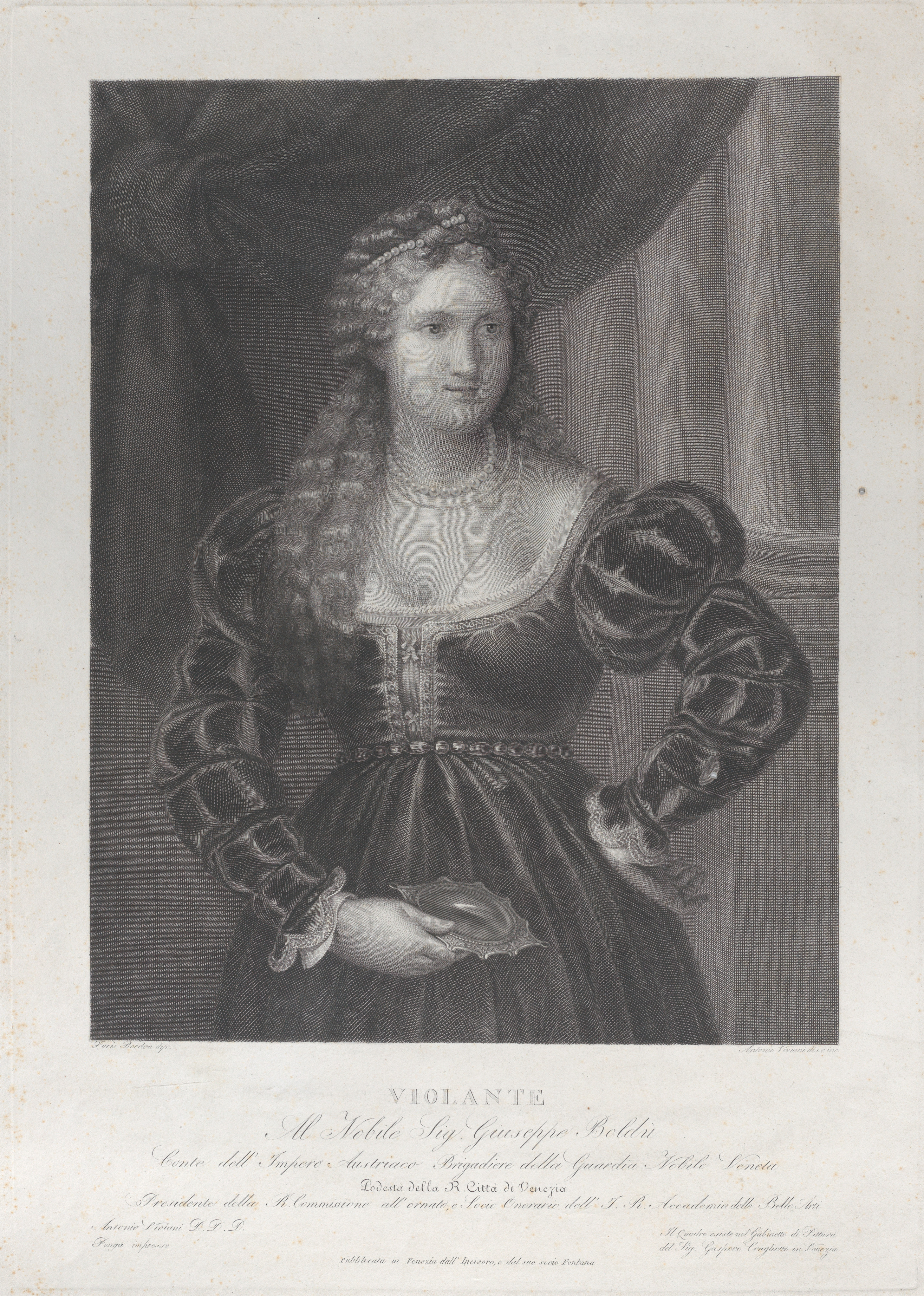A centuries-old black-and-white etching depicts an aristocratic woman from possibly the 1800s. She stands in an opulent setting with heavy drapes and classical columns suggesting a stately home or a theater. The woman, who is distinguished by her wealth, wears an elaborate velvet ballgown featuring puffy sleeves adorned with frills and lace along with a cinched waist highlighted by a belt. Her reddish, curled hair is intricately styled, possibly held with a clip or fashioned into a long braid. She accessorizes with multiple pieces of jewelry, including two pearl necklaces. The woman strikes a stately pose with her left hand akimbo, her forearm resting on her hip, while her right hand holds a metal object—potentially a seashell—resting against her abdomen. Her head is turned to the left. The bottom of the etching displays the small, cursive text "Violante" and "Il Clanti Amia" in Italian, adding a touch of historical authenticity. Despite the monochromatic palette of black, white, and gray, the detailed attire and setting vividly capture the regality and elegance of a bygone era.